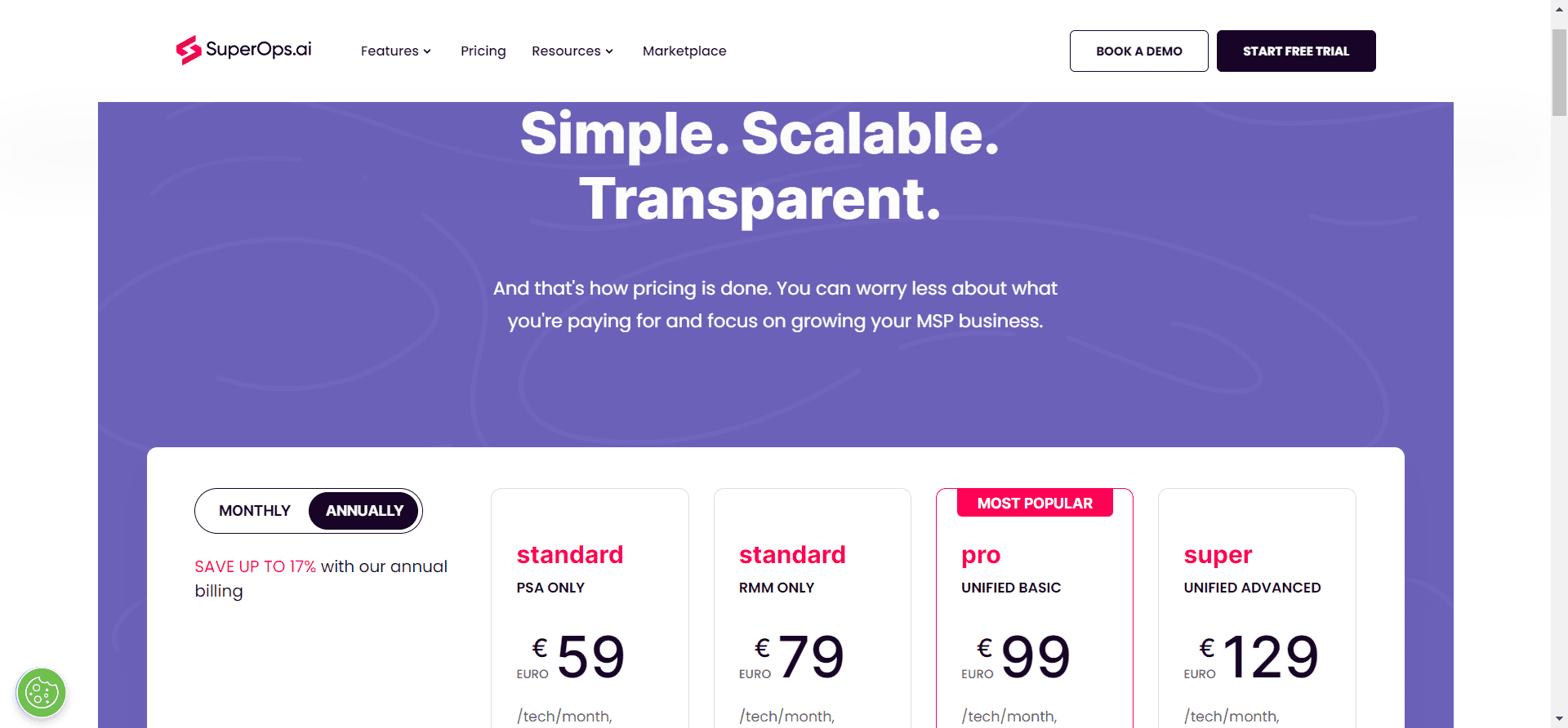This image showcases the subscription page of the SuperOps.ai website. Prominently displayed on the top left is the SuperOps.ai logo, accompanied by a distinctive red line symbol. The website menu features options for "Features," "Pricing," "Resources," and "Marketplace." On the upper right, there are prominent buttons for "Book a Demo" and "Start Free Trial." The page emphasizes a simple, scalable, and transparent subscription model. The available plans include: Standard Subscription (PSA only) for $59, Standard Subscription (RMM only) for $79, Nexus Pro Unified Basic for $99, and Nexus Super Unified Advanced for $129.